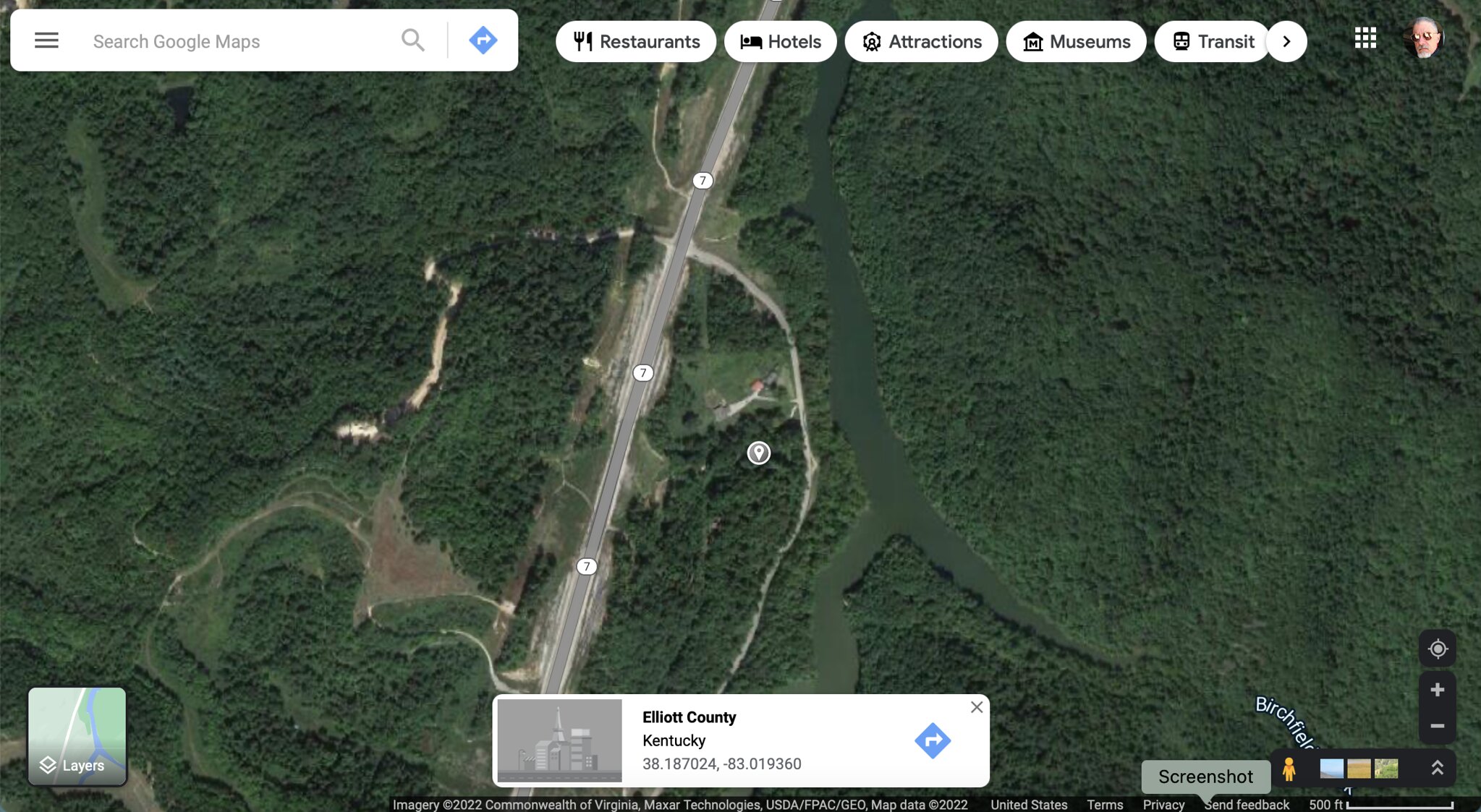A screenshot of a Google Maps interface is prominently displayed, featuring the search bar at the top with the text "Search Google Maps," accompanied by a magnifying glass icon and a blue "Directions" button. Just below the search bar are quick-access buttons labeled "Restaurants," "Hotels," "Attractions," "Museums," and "Transit," spanning across the top of the image. The main view is a detailed aerial perspective showcasing a vast expanse of land densely populated with green trees and foliage. A large, central road bisects the landscape, with various small white markers indicating points of interest or structures. Among these, a solitary house is faintly discernible due to the high altitude of the view. At the bottom of the image, the text "Elliott County, Kentucky" is displayed within a white box, accompanied by a small gray icon.